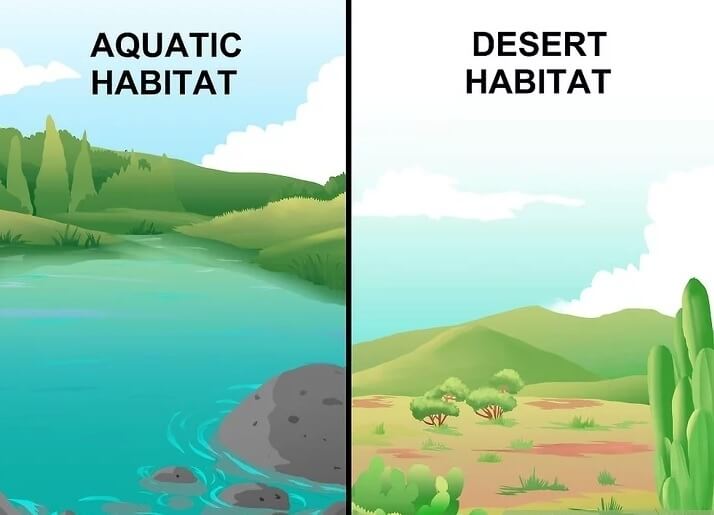This illustration is a comparison graphic, likely designed for a presentation, which is divided down the middle by a thick black line. The left side is labeled "Aquatic Habitat" in black Arial font and depicts a serene lake. In the foreground, small gray rocks and a large boulder emerge from the blue water, while patches of grassy land occupy the middle ground. The background showcases a line of simple, green hills and trees set against a blue sky dotted with white, puffy clouds. The right side is labeled "Desert Habitat," contrasting by featuring a relatively flat landscape with less vegetation. The foreground contains cacti and clusters of grass, while the middle ground has sparse bushes. The background reveals pale green hills or mountains under a similarly blue sky with white clouds. Together, these images effectively contrast the lushness of an aquatic environment with the arid characteristics of a desert landscape.